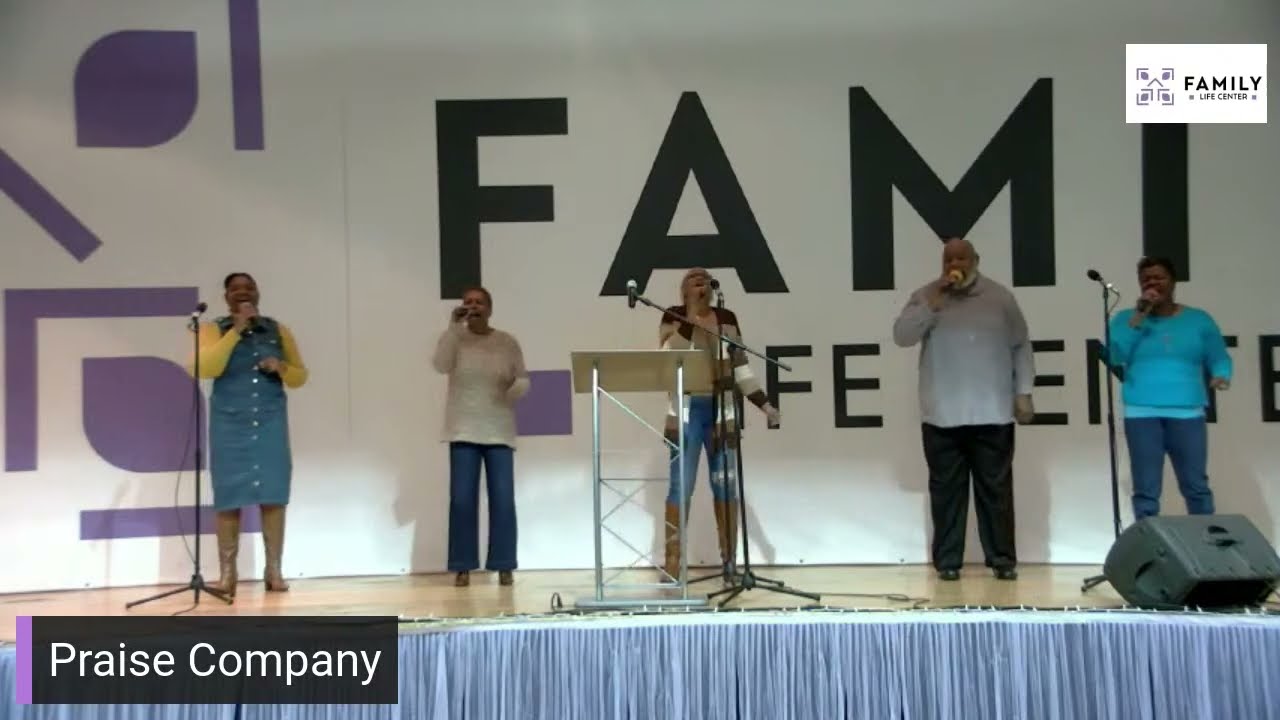The image depicts a group of five casually dressed black individuals performing on a wooden stage. Each person holds a microphone, with three using microphone stands placed in front of them. They stand behind a small music stand and a black monitor sits in the lower right-hand corner of the stage. The stage is adorned with gray bunting and features a backdrop with a large white sign displaying the partially visible text "F-A-M-I," suggesting the word "FAMILY." Additional letters, "F-E-E-N-T" and possibly the beginning of another character, are obscured by the performers. The background includes purple symbols resembling an abstract design with a leaf and geometric shapes. On the bottom left of the image, a black box with the white text "Praise Company" is present. The individuals' attire includes: a yellow shirt with a denim button-up, a tan sweater with jeans, a vest with jeans and cowboy boots, a gray button-down shirt with black pants and black shoes, and a blue sweater with jeans. An amplifier is also visible on the stage.